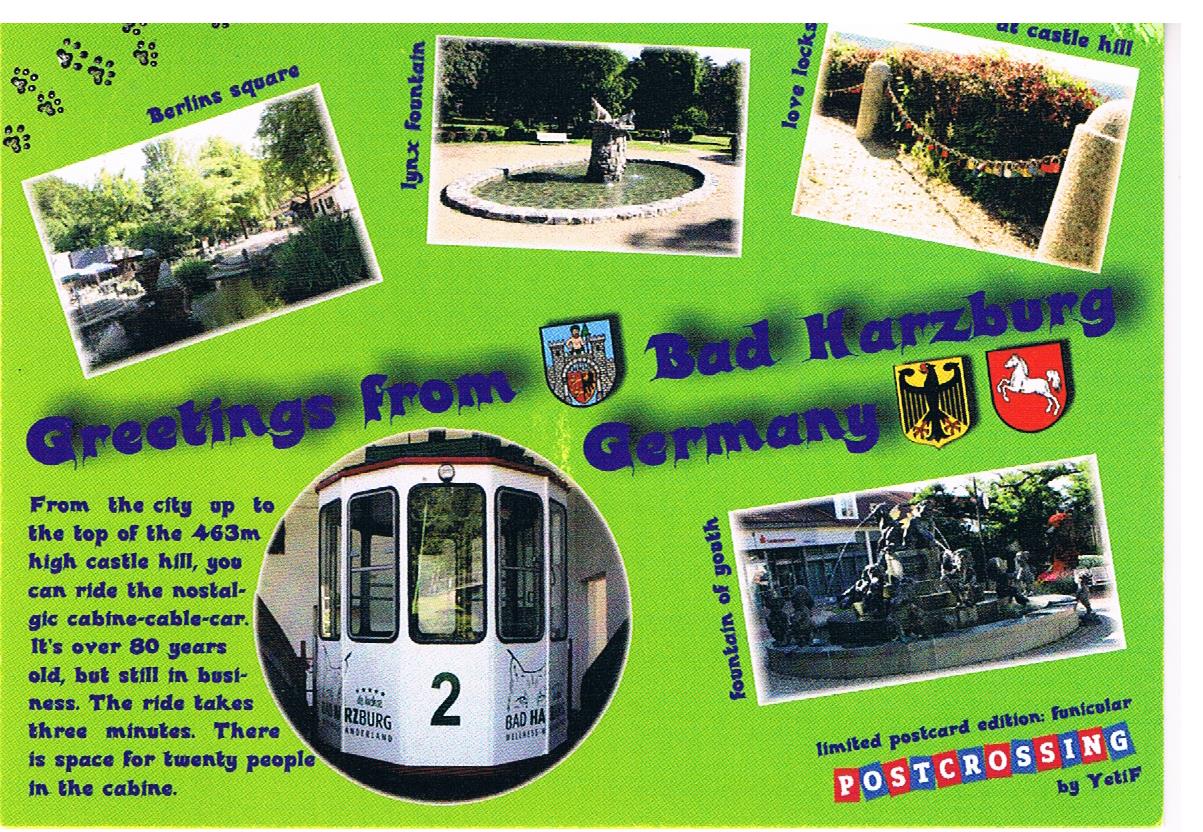This vibrant postcard features a bright lime green background and prominently reads, "Greetings from Bad Harzberg, Germany." The postcard is accented with three main images, each accompanied by captions. The first image, titled "Berlin's Square," showcases a picturesque canal or pond flanked by quaint buildings and an open area. The second picture is labeled "Link's Fountain," depicting a fountain made of stone or concrete, with water surrounded by architectural elements. The third image illustrates two stone pillars adorned with love locks, adding a charming touch to the scenic vibe.

Above these images, blue text commemorates each sight, and below them, a tram image is highlighted with an intriguing note about the nostalgic cabin cable car that ascends to the 463-meter high Castle Hill. Further details mention that this cabin has been in operation for over 80 years. Completing the postcard, the bottom right corner contains the words, "Limited Postcard Edition" and "Post Crossing by Yotif," with an overlay of playful paw prints adding a whimsical note. Collectively, these elements create a rich, detailed tapestry of Bad Harzberg's enchanting locales and historical layers.